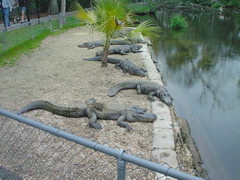This small, square color photograph captures a gravelly area adjacent to a murky, greenish body of water, possibly a pond or swamp. The water is bordered by a paved concrete edge. Prominently, the image features a row of five long, slender, grayish alligators with very long tails and snouts, arranged from the top to almost the bottom of the photo. These alligators are resting, with one closest to the viewer facing the water, and another appears to be entering it. A blue railing runs diagonally across the foreground, while the background shows a mix of greenery, including some miniature palm-like trees and a tall chain-link fence. There is blurred greenery, likely a tree, with palm-type leaves in the upper right corner. The setting is close to a public walkway, noticeable for casual pedestrian activity, including a man and a woman walking, and another person on a scooter, illustrating the proximity of people to the alligators.